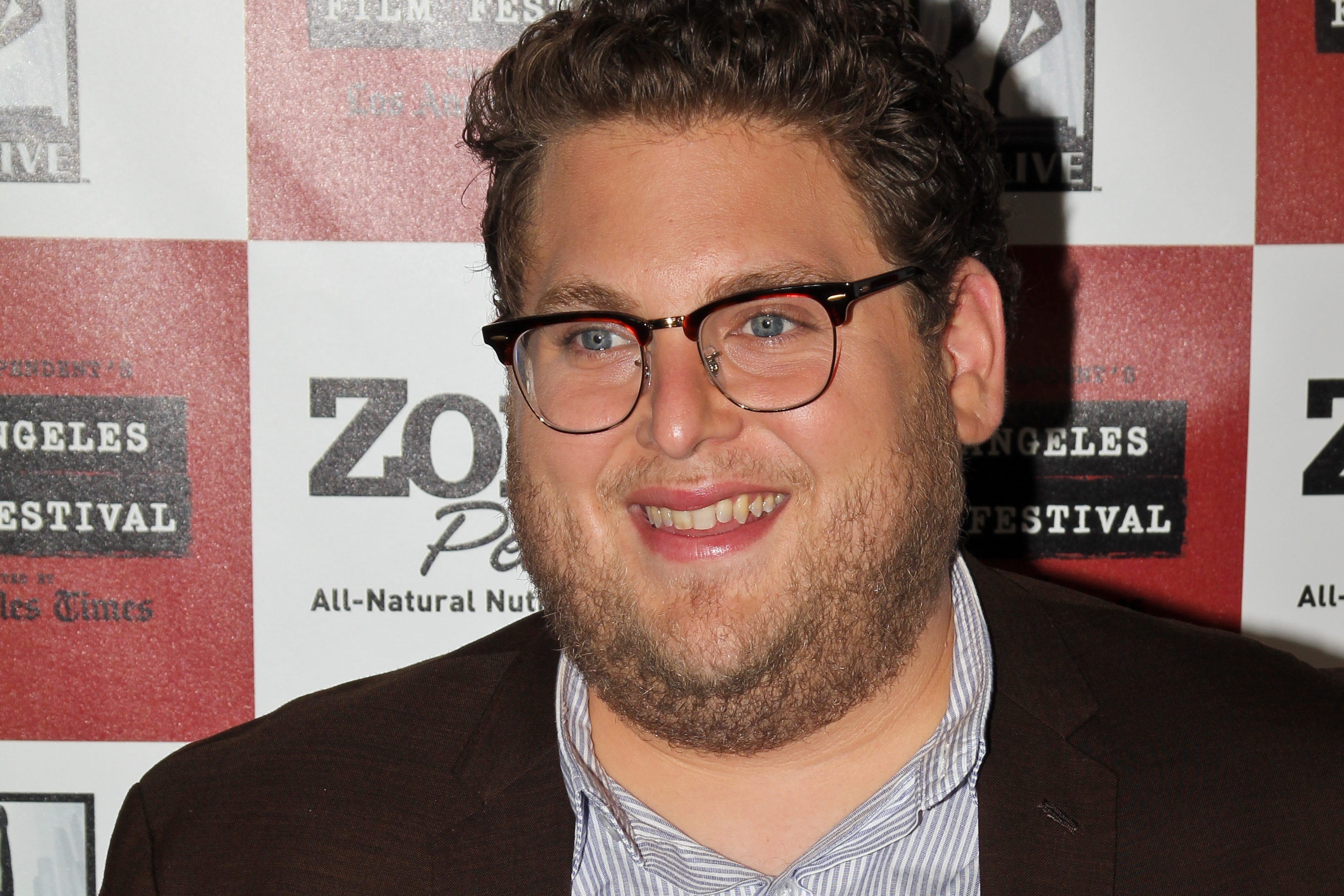The image features actor Jonah Hill smiling at the camera while attending the Los Angeles Film Festival. Hill, known for his chubbier physique and double chin, is dressed in a black suit jacket over a white and gray striped shirt. He sports medium-length curly dark brown hair, a black beard, and vintage-inspired glasses with black acetate on the top and wire frames underneath. His blue eyes are clearly visible behind the glasses. The background prominently displays a white and red checkered banner adorned with multiple logos and advertisements for the festival, though some of the text is obscured. The photograph focuses on Hill from the shoulders up, placing him centrally against the event backdrop.